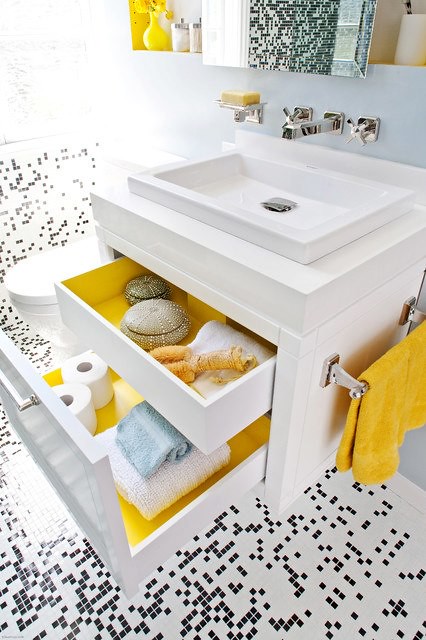The image depicts the interior of a modern bathroom with a cohesive color scheme that emphasizes yellow accents. A prominent white bathroom cabinet, featuring two drawers with vividly painted yellow interiors, stands out in the scene. This bright yellow matches a towel neatly hanging on a towel rack affixed to the side of the cabinet. Atop the cabinet rests a sleek, square-shaped sink with chrome faucets extending stylishly from the wall. Above the sink is a sliding mirror, which reveals a medicine cabinet filled not with medicine, but with white and yellow beauty products. The bathroom's floor is adorned with a tiled pattern of small white and black squares, adding a crisp contrast to the overall design.